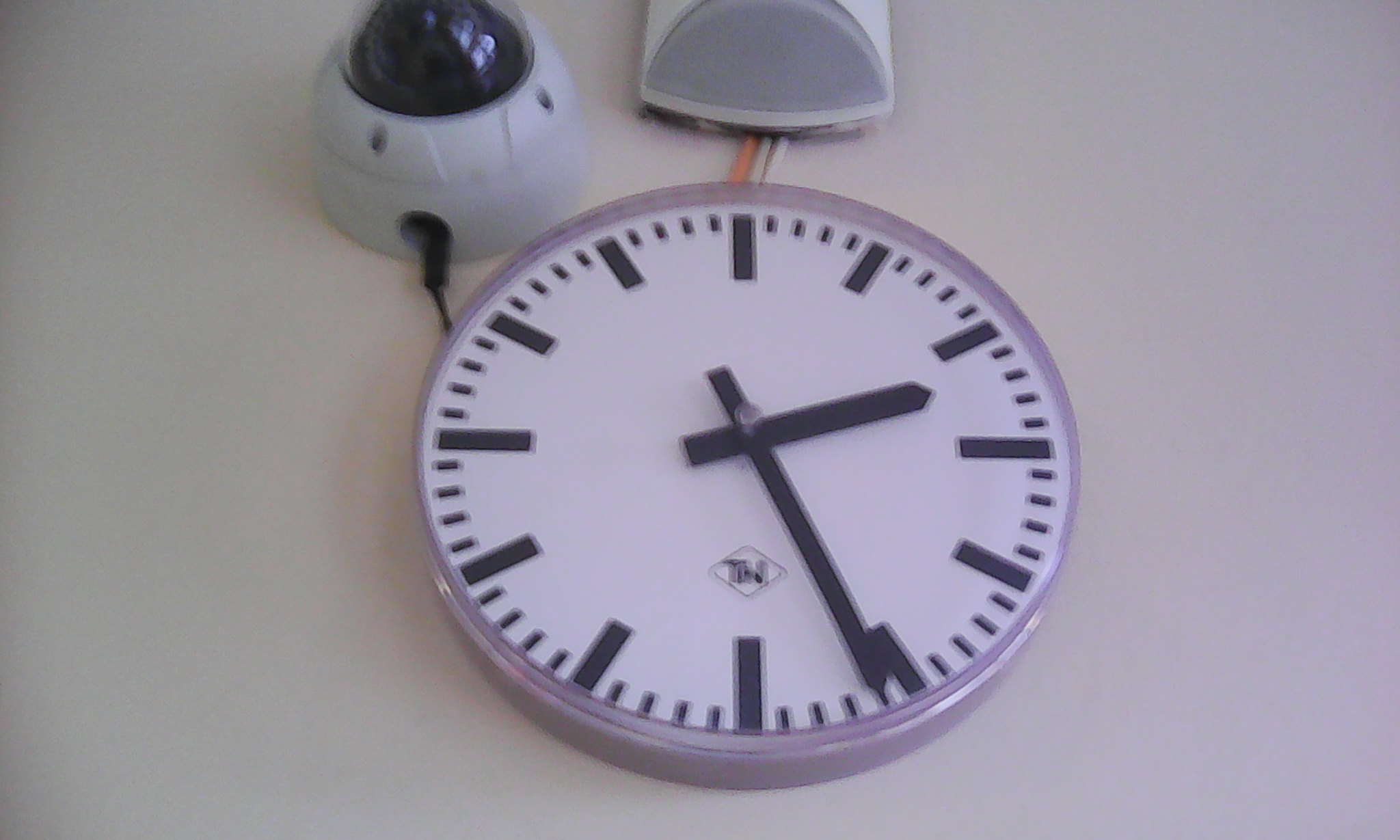The image features a contemporary round-faced clock with minimalist lines in place of numerical markers, giving it a modern yet elegant appearance. The clock hands are positioned to indicate the time as 3:30. Attached to the clock is a cable that connects to a separate, spherical white device, which appears to serve as an advanced alarm system. This device includes a transparent dome, suggesting it may light up when activated. Additional wires extend from this alarm unit to a speaker, designed to enhance the alarm's sound, ensuring it is audible even from a distance. The clock is branded with the initials "TIW" discreetly placed in the lower corner, signifying its maker.